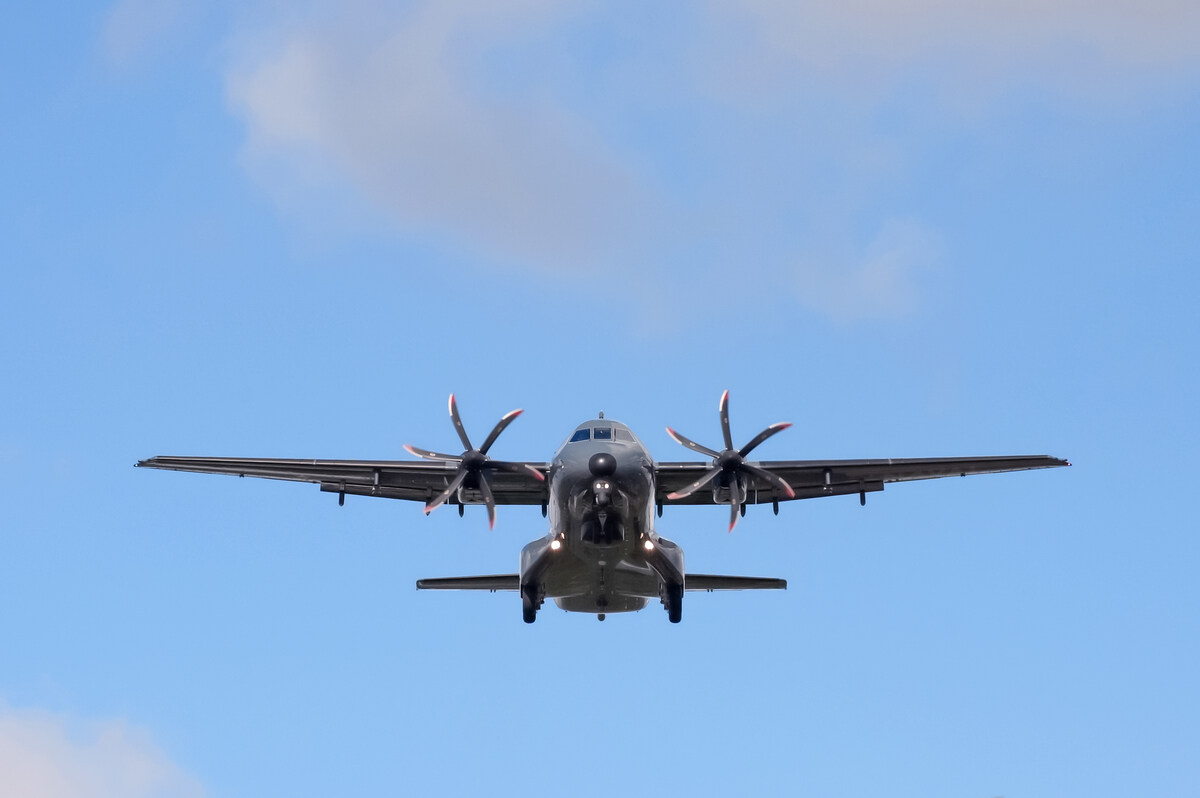The image shows a dark gray airplane flying in a clear, blue sky with a few scattered, wispy clouds. One small cloud is positioned just above the plane, and another smaller cloud is to the bottom left. The airplane, possibly a military aircraft, is seen from a front and slightly below angle, showcasing its streamlined design with two stationary propellers at the very front, each having six sharp blades. The nose of the plane is black, contrasting with the dark gray body. The plane has one main wing and a tail wing, and two sets of lights at the front: one spanning the width of the airplane’s body and another limited to the nose. The cockpit features three visible windows. The background is otherwise entirely clear, emphasizing the aircraft as the central focus of the picture.